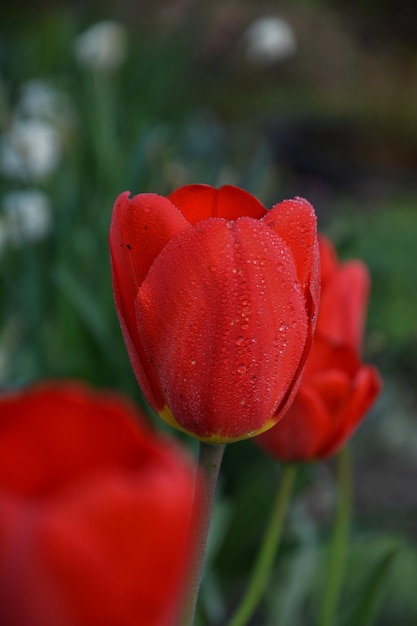The photo is a close-up shot of three reddish-pink tulips, with the central tulip in sharp focus. This tulip, with its robust stem and light green base, appears to be freshly kissed by early morning dew, displaying delicate drops of water clinging to its petals. The background is beautifully blurred, accentuating the primary tulip's striking colors. In the backdrop, hints of green foliage and clusters of white flowers can be seen, contributing to a lush, natural setting. The other two tulips on either side are out of focus, adding depth to the image while allowing the main tulip to stand prominent and radiant in the foreground.